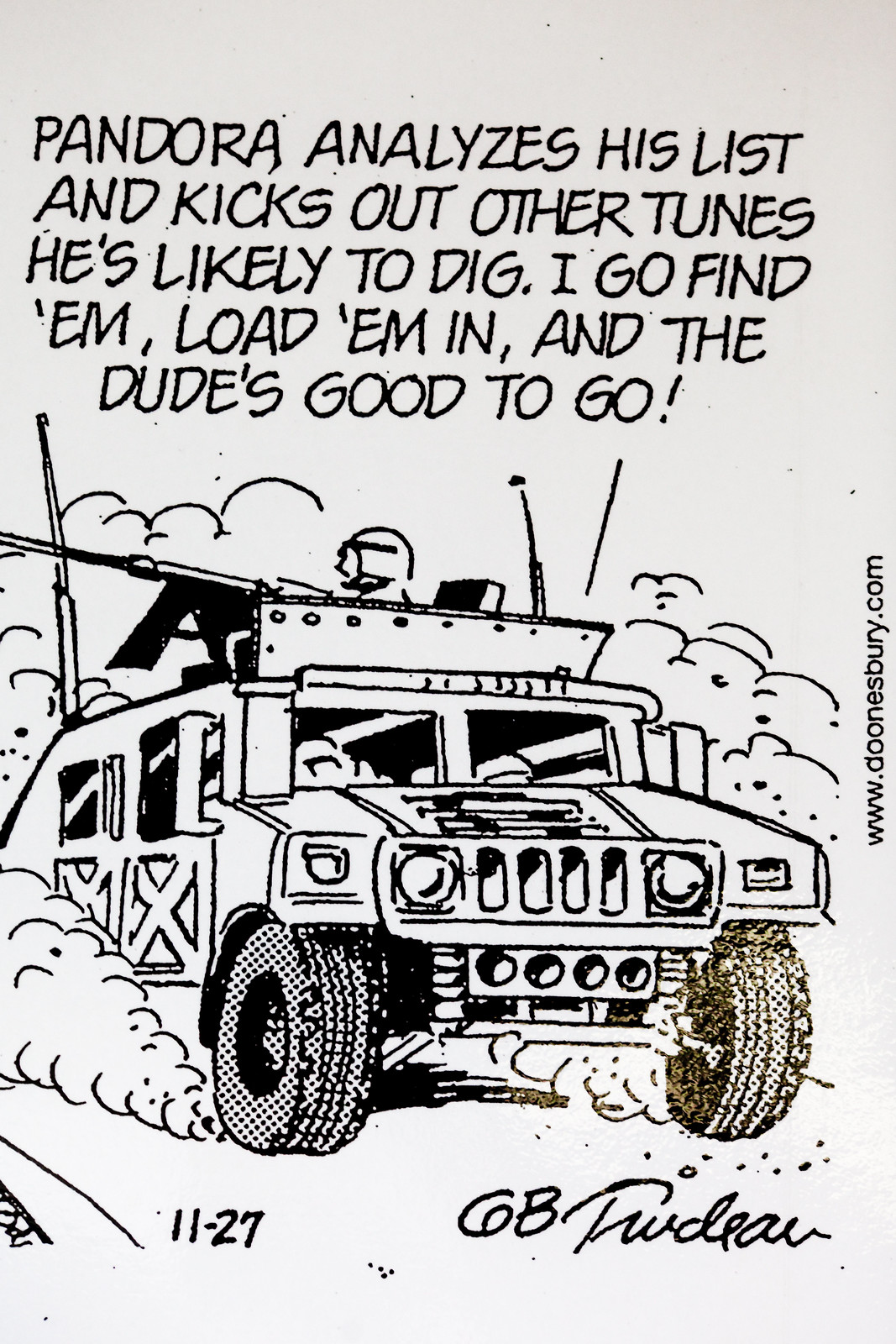The image is a single-panel black-and-white comic created by GB Trudeau, dated 11-27, depicting a cartoonish military tank against a white background. Emerging from the turret at the top of the tank is a soldier aiming a sniper rifle. Behind the vehicle are clouds of smoke trailing it. At the top of the panel in capital black letters, the words read, "PANDORA ANALYZES HIS LIST AND KICKS OUT OTHER TUNES HE'S LIKELY TO DIG. I GO FIND THEM, LOAD THEM IN, AND THE DUDE'S GOOD TO GO!" The illustrator's signature, GB Trudeau, is located in the bottom right corner, and the very right-hand side of the image includes the website, www.doonesbury.com.